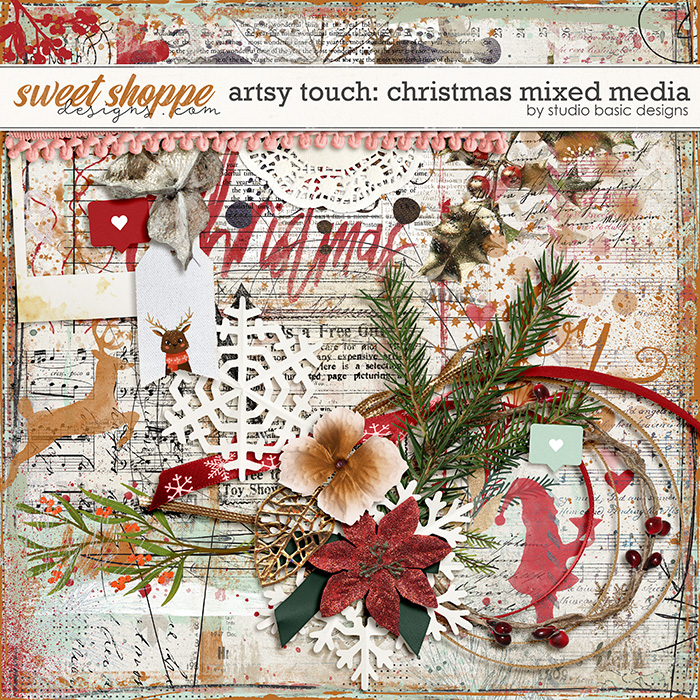The image showcases a richly detailed Christmas collage, accentuated with a vibrant amalgamation of festive elements arranged thoughtfully on a background of assorted scraps of paper. Prominently featured are two white hearts – one set against a red background and another on an olive backdrop – symbolizing holiday sentiment. A striking red flower and a brown flower lie centrally amidst green ribbons and leaves, including a gold and fern leaf, adding texture and depth. 

Additionally, a cut-out snowflake and a reindeer enhance the wintry theme, while strings adorned with red beads form a circular pattern, and a delicate lace doily peeks in from the top of the collage. Red berries and red words spelling "Christmas" are scattered around, blending with the overall festive ambiance. 

The top of the image is bordered by a pale strip or banner with the text "Sweet Shoppe" in orange and "Artsy Touch: Christmas Mixed Media" in black, followed by the artist's signature - "by Studio Basic Designs," in a smaller black font. These elements, coupled with music notes and various decorative touches like red and green holly sprigs, complete the collage's traditional yet dynamic Christmas aesthetic. The composition is rectangular, potentially serving as a Christmas card, postcard, or an advertisement for a shop named "Sweet Shoppe".